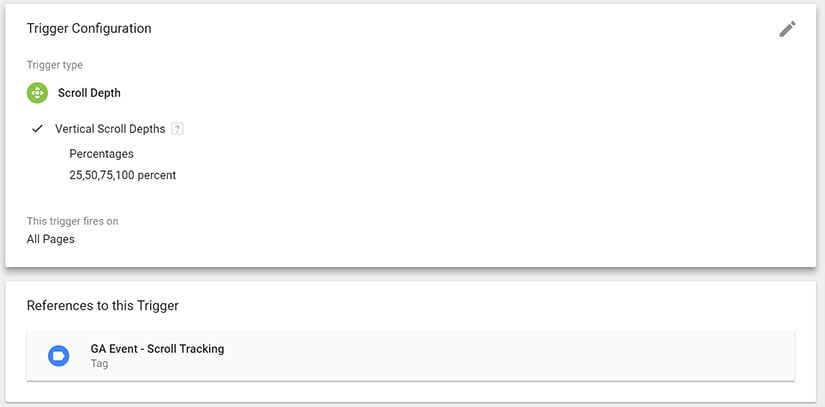The image depicts a section of a web page or app interface with a clean, white background.

**Top Left Corner:**
- The heading "Trigger Configuration" is displayed in a black font with both 'T' and 'C' capitalized.
- Directly beneath this heading, the text "Trigger Type" appears in a faded or grey font, where "Trigger" starts with an uppercase 'T' while "type" is in lowercase.

**Below "Trigger Type":**
- A green icon with a diamond shape enclosing a circle is present.
- Next to the icon, the words "Scroll Depth" are written in a black font, with both 'S' in "Scroll" and 'D' in "Depth" capitalized.
- A checkmark is placed beside the text "Vertical Scroll Depths."
- Indented beneath "Vertical Scroll Depths," the percentages "75, 100%" are listed.

**Further Down:**
- A slight gap separates the next section, which begins with the text "Trigger Fires On" in a faded grey font.
- Below this, in a bold font, the words "All Pages" are displayed.

**Top Right Corner:**
- An icon that signifies the option to edit the page is visible.